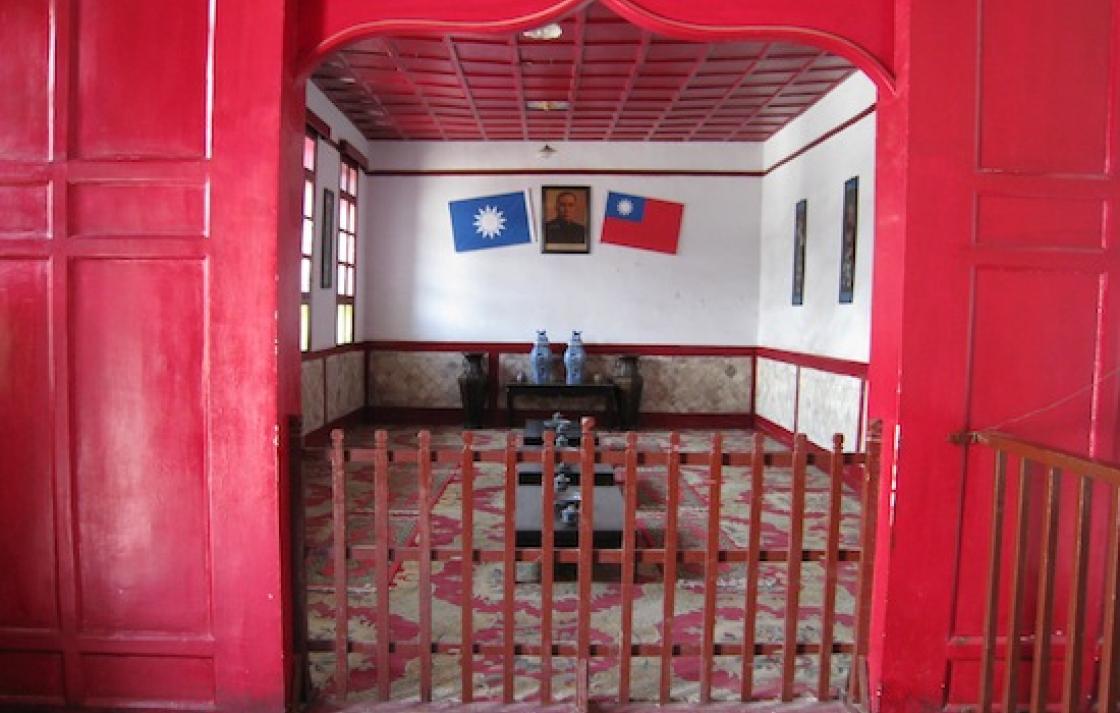The photograph captures an elaborately decorated private dining hall styled in traditional Japanese aesthetics. The walls facing the viewer are painted in a rich red hue, giving the space a distinct, warm ambiance. At both ends of these red walls, there are intricately textured wooden gates that create a barrier, possibly indicating the room is part of a museum exhibit.

Inside the hall, the far wall is predominantly white with red trim, adorned with two flags. The left flag is blue with a white sun in the center, while the right flag is red with a blue rectangle in the upper left quadrant, also featuring a sun. Between these flags, a framed portrait of a dignified man, possibly a military leader or general, is prominently displayed.

Directly below the portrait, a bench holds two blue vases, adding to the room's traditional decor. The floor is covered with a red and gold carpet that has a floral pattern, enhancing the room’s elegance. In the center of the carpet, there are three low black tables, each set with various teapots, bowls, and plates, indicating this could be a dining setup where guests would sit on the floor to eat in true Japanese style. The combination of these elements not only emphasizes the cultural richness of the space but also lends an air of exclusivity and historical significance.